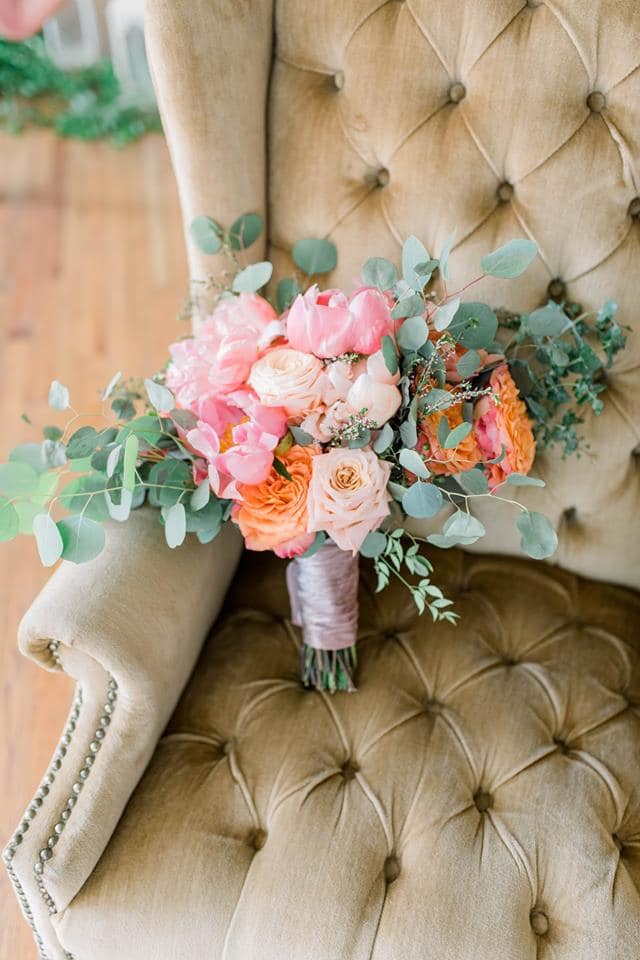In the photograph, a vibrant bouquet of flowers is elegantly draped over the corner of a tan, button-tufted chair, with one of the armrests partially visible. The bouquet, comprising predominantly roses, showcases a vivid array of colors including pink, light pink, white, orange, and purple. Intermingled among the roses are various other plants, adding lush greenery to the arrangement. The bouquet is tightly bound in the middle with a wrapping that resembles a pink lanyard, while some clear plastic wrapping can be seen at the bottom, allowing several stems to poke through. The floral arrangement leans against the armrest, suggesting a casual yet purposeful placement. The chair appears to be set against a wooden floor, with hints of additional floral elements in the background. The photograph is taken from a standing position, looking down at the bouquet, emphasizing the intimate and cozy setting. The neutral tones of the chair contrast beautifully with the vibrant colors of the flowers, creating a visually appealing and detailed composition.